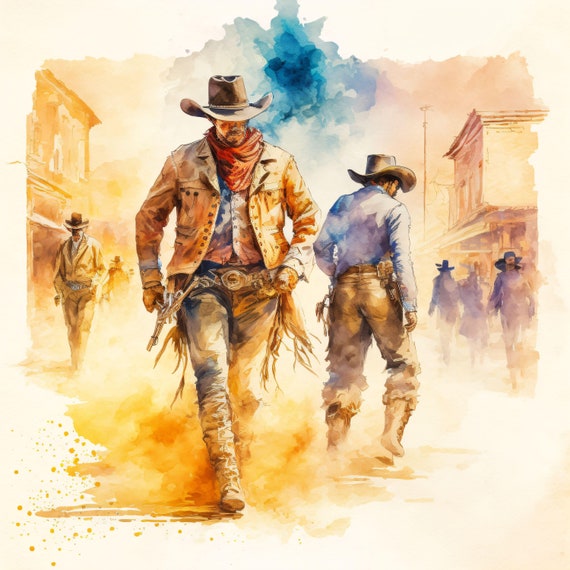This vibrant watercolor painting vividly captures an old country and western scene, characterized by its fluid and slightly stylized appearance. Dominating the foreground, a cowboy strides towards the viewer; his eyes obscured by the brim of his large black hat. He wears a red bandana around his neck and a coat over his shirt, complemented by chaps and faded blue jeans tucked into his high boots. Beside him, another cowboy, clad in a blue shirt and dark pants, walks away, his back turned to the viewer. The scene suggests the anticipation of a standoff, adding an air of tension and drama.

In the mid-ground, the painting features loosely depicted figures and classic western buildings on either side, enhancing the historical ambiance. The background is dominated by a flowing swatch of blue that represents the sky, while beneath it, an orange sprawl evokes the ground, these being the painting's most striking color elements. The watercolor medium infuses the scene with a hazy, dreamlike quality, characteristic of the genre's fluidity and blending colors. The overall effect is a blend of realism and stylization, making the piece both striking and evocative of the wild west.